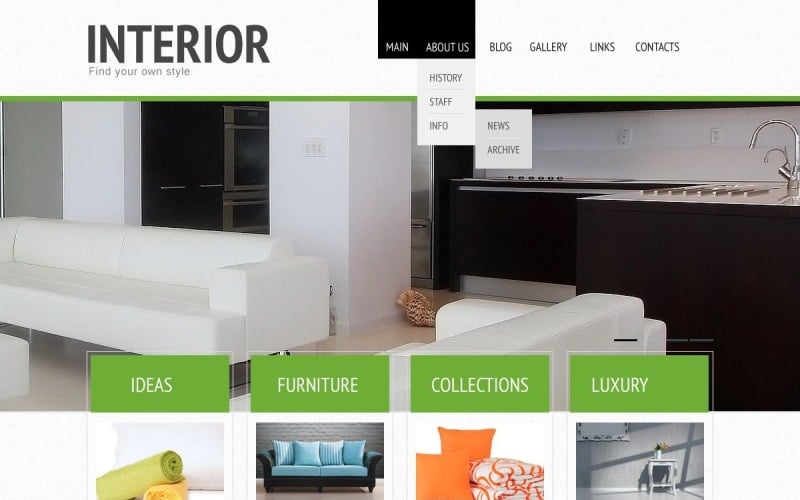In this webpage, the top left corner prominently displays the name of the website. To the right, a navigation bar features various labels or links, including "Main," "About Us," "History," "Staff," "Info News," "Archive," "Zee Blog," "Gallery," "Links," and "Contacts." Below this navigation bar, additional sections labeled "Ideas," "Furniture," "Collections," and "Luxury" are visible. The main image on the page showcases a modern living room scene with a sleek white couch in the foreground. In the background is a stylish kitchen area. The overall color scheme of the layout includes shades of green, white, and black. Notably, a decorative snail shell sculpture is visible in the background, adding an artistic touch to the setting.